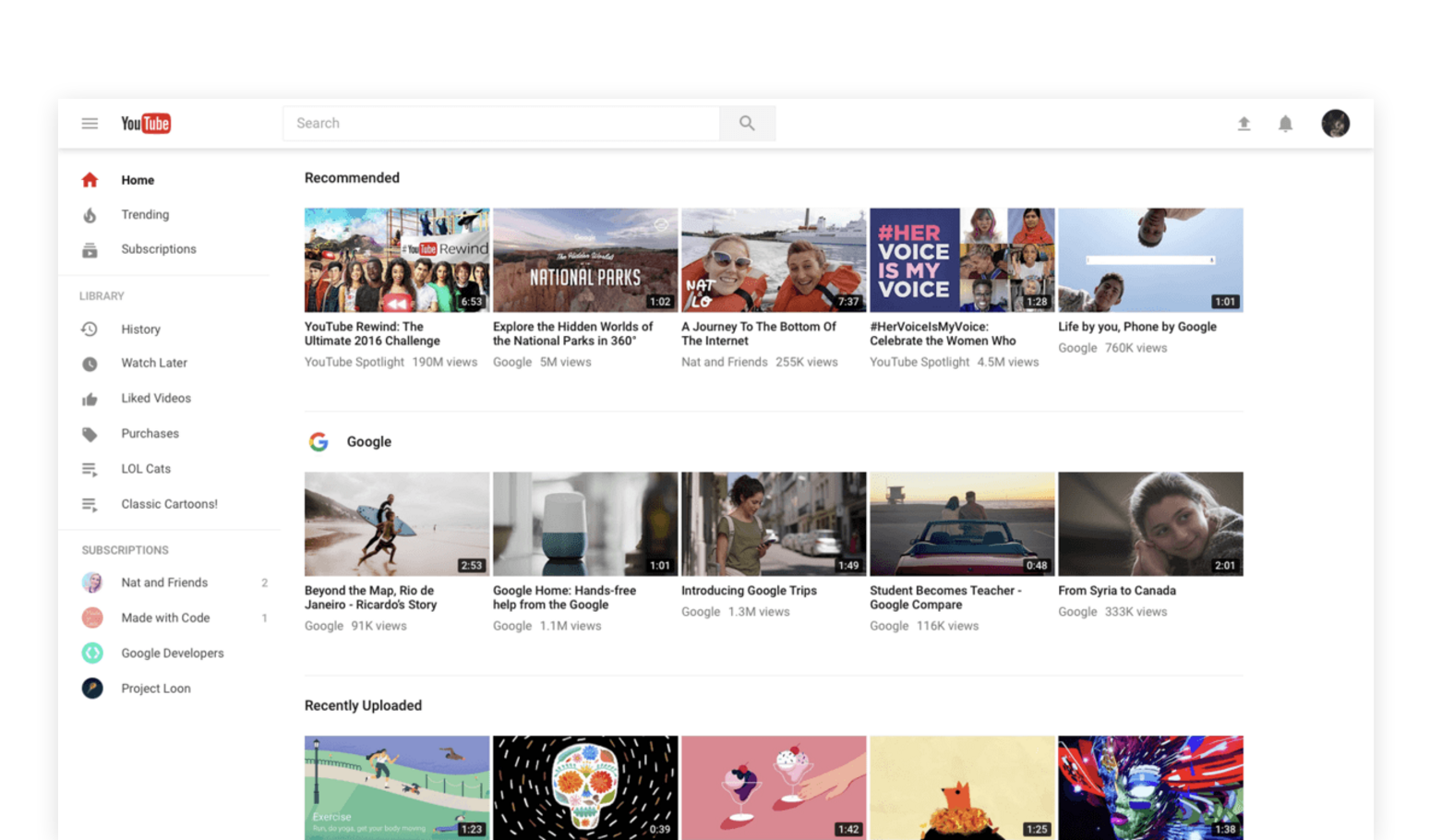This image is a screenshot of the YouTube homepage. In the upper left corner, the YouTube logo is prominently displayed with the recognizable red 'play' icon surrounding the white 'tube'. The left-hand sidebar features options such as 'Home', 'Trending', and various other selections for easy navigation. At the top center, there is a search bar where users can type in queries to find specific content.

On the right-hand side, notification alerts are visible, likely indicating new updates or messages. The central part of the screen displays a section titled 'Recommended', with video suggestions tailored to the user's preferences. Among these suggestions are a video titled "YouTube Revealed" and a challenge video from 2016. Another recommendation titled "National Parks: A Journey to the Bottom of the Internet" features an image of two people on a boat. Additional video titles like "Her Voice is My Voice" are present, alongside various other tailored video recommendations.

Further down, there is a category labeled 'Recently Uploaded', which shows images of YouTube videos that have recently been uploaded by others or by the user themselves, providing quick access to the latest content.